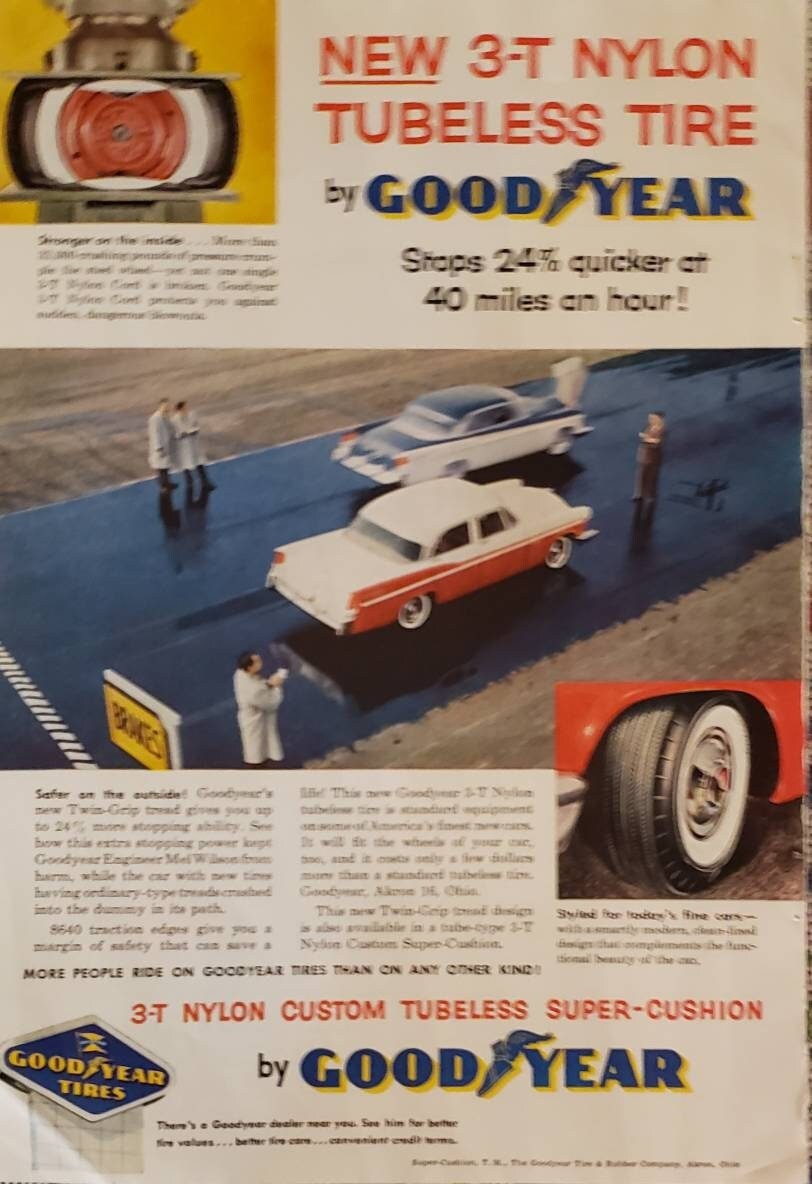This vintage color print advertisement for the Goodyear "New 3-T Nylon Tubeless Tire" features a blend of illustrations and photographs, painstakingly detailed and structured in a portrait orientation. At the top right, prominent red text excitedly announces the product, paired with the iconic Goodyear logo. The headline is reinforced by a subtitle asserting that these tires stop 24% quicker at 40 miles per hour. 

To the upper left, an illustration elucidates the tire's construction, possibly showcasing a tire pressure test where the tire is being compressed by a machine. The middle section commands attention with a full-width illustration depicting a racetrack scene. Here, several men in white lab coats carefully observe two vintage automobiles halted side by side at an angle, with the assumption being that the red car, equipped with the Goodyear tires, stopped sooner than the blue car.

On the lower right, there is a close-up photograph of the tire fitted on a mostly cropped-off red car, accentuating the tire's tread and build. Across the bottom, a vibrant red banner boldly states "3-T Nylon Custom Tubeless Super Cushion," flanked by additional Goodyear logos. To the lower left, the ad concludes with a dark blue Goodyear tire sign with yellow lettering, reinforcing brand identity.